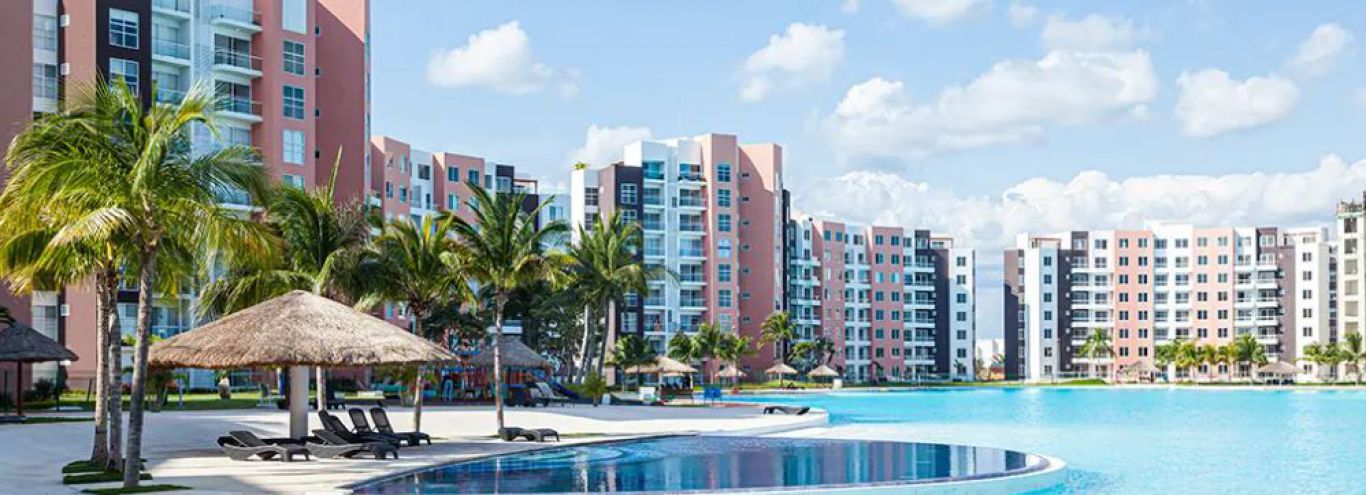The photograph captures a luxurious resort area featuring pristine blue water that is exceptionally clean and clear. In the foreground, there's a cabana with a thatched roof providing shade over numerous black lounging chairs. This relaxing spot is surrounded by tall, lush palm trees with green fronds and brown trunks. A large swimming pool, with a possible hot tub elevated above the main pool area, stretches out and dominates the scene. In the background, a series of tall buildings, presumably hotel rooms, extend across the skyline. These buildings are primarily brown and white with hints of pink and blue, likely due to shadow. They appear to be part of the same complex and vary in height. The vivid blue sky is adorned with fluffy white clouds, adding to the serene atmosphere of this idyllic outdoor setting.